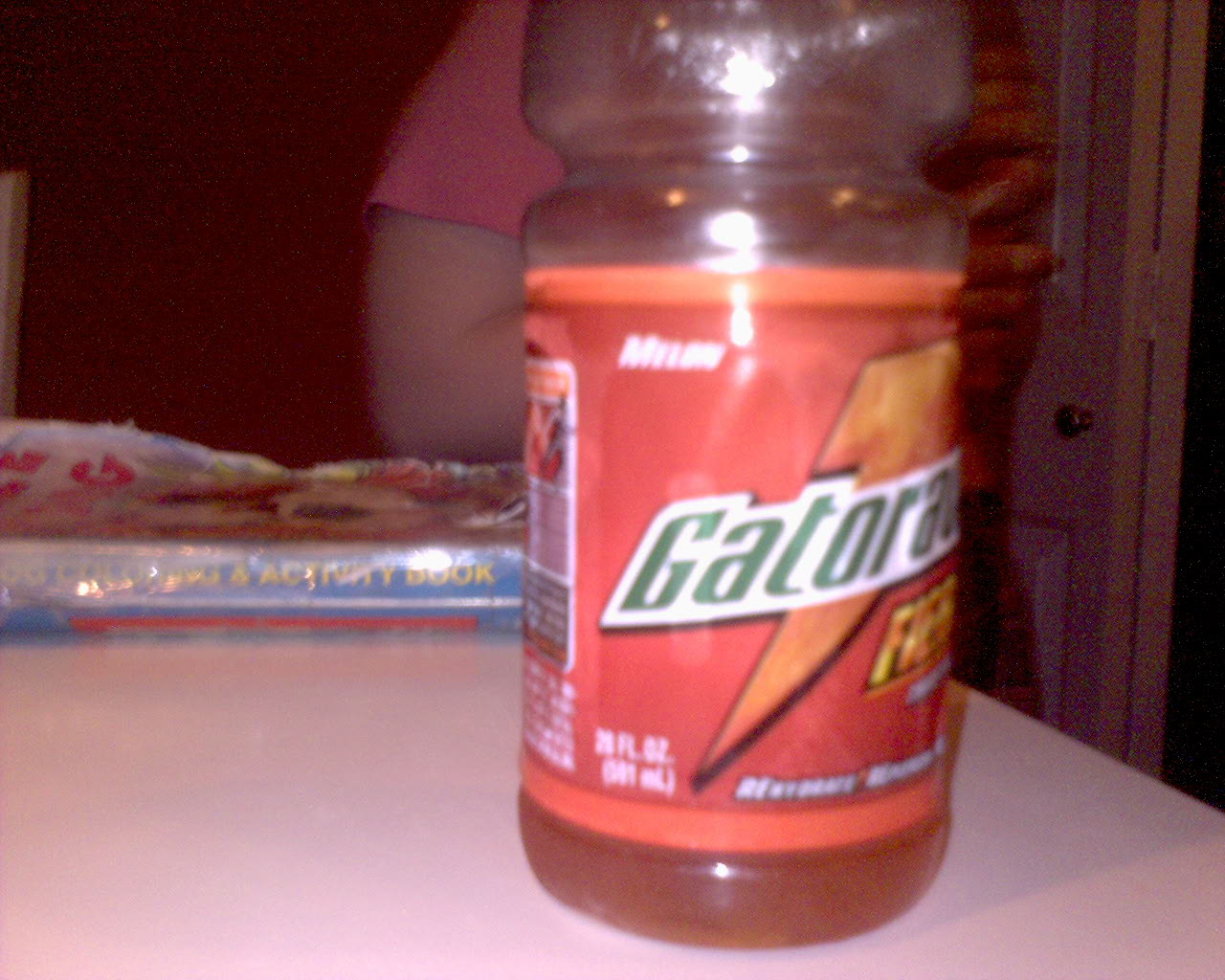This image prominently displays a slightly blurred Gatorade bottle positioned center-right on a white table. The bottle, which is made of plastic, contains an orange liquid and features an orange lightning bolt along with the word "Gatorade." The label also includes the word "fierce," suggesting a specific flavor variant, possibly melon. The bottle is about half-empty, with some liquid visible at the bottom. In the background, a person wearing a peach or pink short-sleeved t-shirt is partially visible, with their upper arm and fingers slightly in view. Behind the Gatorade bottle, there is a book that resembles a child's activity book, identifiable by its blue border, cartoon characters, and text that appears to describe it. The image overall is slightly out of focus, complicating the clarity of finer details.